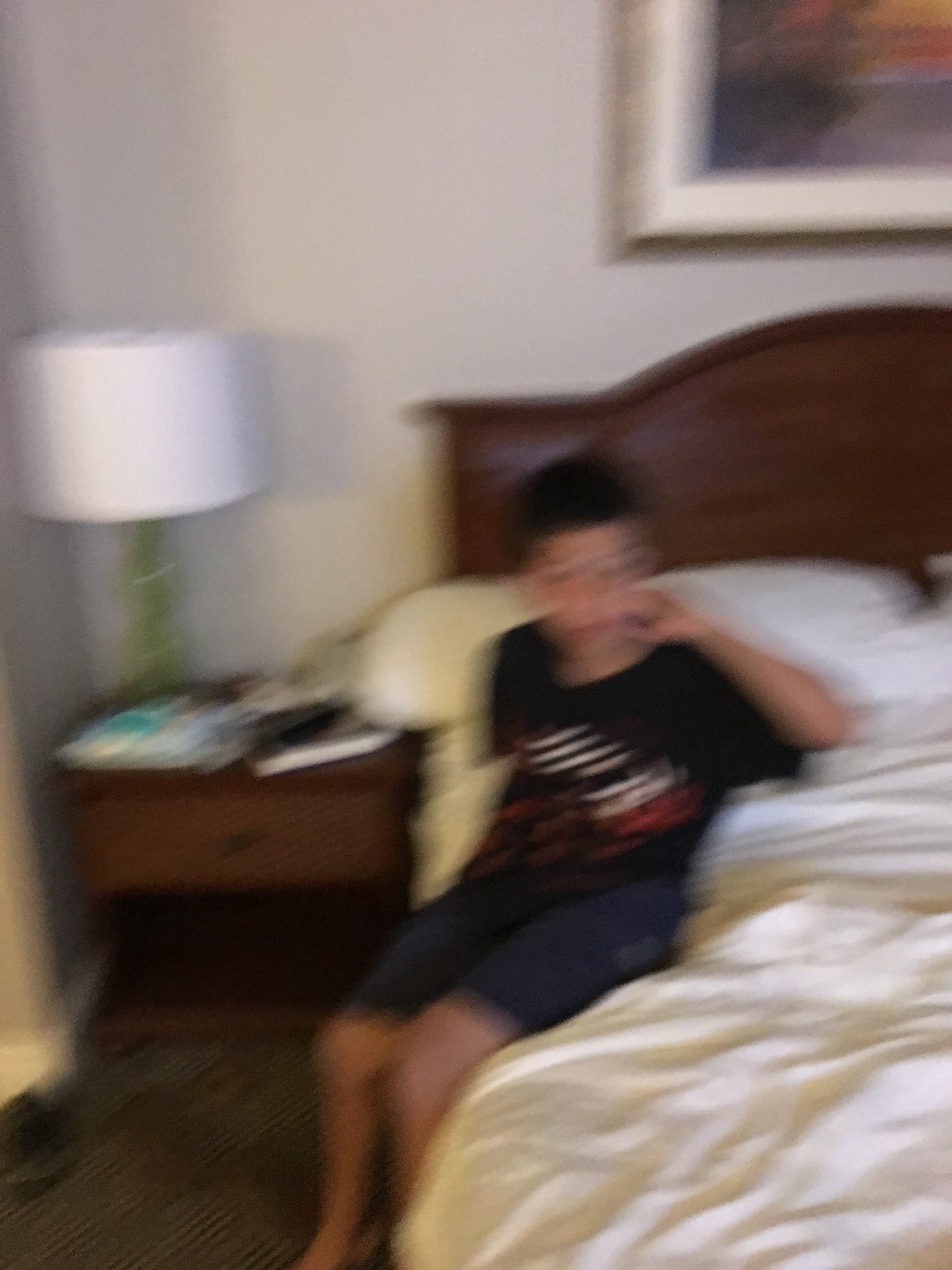In this very blurry photograph, a boy with short brown hair and glasses is captured sitting on the edge of an unmade bed, possibly just waking up. He is dressed in a black t-shirt with white markings and blue shorts. One of his hands is raised to his face, while the other seems to be resting behind him. The bed is covered with white sheets and has a white pillow, contrasting with the dark brown wooden headboard. The bedroom features gray walls, and there is a partially visible picture frame with brown and white borders on the wall above the headboard. To the left of the bed sits a wooden nightstand cluttered with books and other miscellaneous items, topped with a green lamp with a white lampshade. Adding to the cozy ambiance, a glimpse of grayish carpet can be seen at the boy's feet.